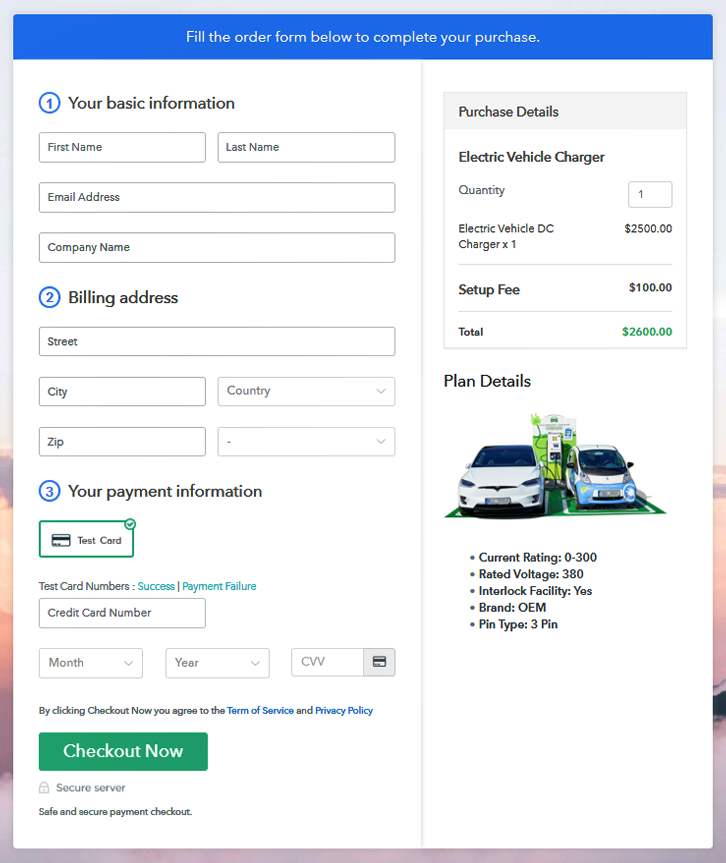This image depicts a checkout page from a mobile app or a website dedicated to purchasing an electric vehicle charger. The layout is organized into a sequence of detailed steps for completing the transaction. 

At the top of the page, a blue bar features a prominent white text instruction: "Fill the order form below to complete your purchase." 

Step one, marked by a blue circle containing the number one and the text "Your Basic Information," is positioned on the left. This section includes input fields for first name, last name, email address, and company name.

Step two, identified by a blue circle with the number two and titled "Billing Address," provides fields for entering street, city, country, zip code, and a placeholder for a telephone number.

Step three, denoted by a blue circle with the number three and labeled "Your Payment Information," includes an illustrated icon resembling the back of a credit card. This step is encapsulated in a green rectangular box featuring a circled checkmark in the upper right corner. It contains text such as "Test Card" and "Test Card Numbers." Adjacent to this, a green label indicates "Success, Payment Failure," despite the contradictory phraseology.

Below these sections, fields are available to input credit card number, expiration month and year, and CVV. A notice below these fields states, "By clicking checkout now, you agree to Terms of Service and Privacy Policy," with the latter terms highlighted in blue.

Further down the page, a green box with white text bears the phrase "Checkout Now." Beneath that, phrases "Secure Server" and "Safe and Secure Payment Checkout" are displayed. 

To the left, under the "Purchase Details" heading, the specifics of the purchase are listed: Electric Vehicle Charger - 1 unit priced at $2,500, and a setup fee of $100, leading to a total amount of $2,600, which is highlighted in green.

Finally, the "Plan Details" section at the bottom includes an image of two cars charging, accompanied by descriptive details about the plan.